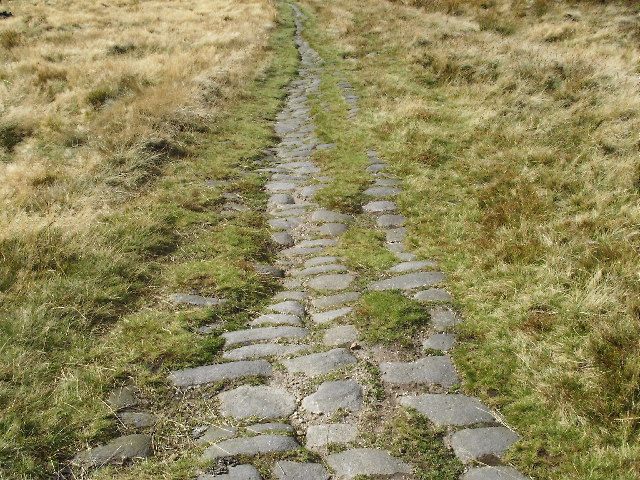The image depicts an overgrown stone pathway embedded in a grassy field, which used to be a full pathway but has since become partially obscured by grass over time. The path comprises handmade stones that are laid out in a random, non-ordinal fashion, with grass growing between many of them. The pathway cuts through a grassy area, where the grass on both sides of the stones is mostly alive and green, though it transitions to a dying, brown hue further away from the path, especially noticeable on the left side. The stones themselves are mostly a cold bluish-gray, with some appearing in a cold gray shade, particularly three stones positioned on the front left end. The scene is brightly illuminated by heavy sunlight, indicating that it is taken during daylight hours.